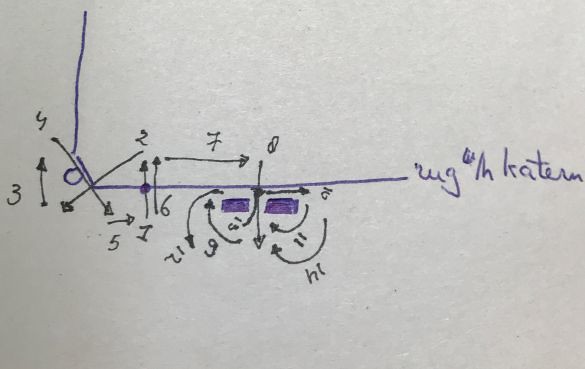The image depicts a complex, intricate formula meticulously written in a combination of black and purple ink. The mathematical notation appears highly advanced and may be indecipherable to those without specialized knowledge. On the right-hand side, a signature, which could possibly read "W-G L-H K-A-T-E-R-N," suggests the author's identity, though the characters might not entirely be Latin letters. The formula features various numbers written exclusively in black ink. Intertwined within the writing are two fully shaded purple rectangles and a hollow circle on the left side, also in purple, adding unique graphical elements to the otherwise text-dominant composition.